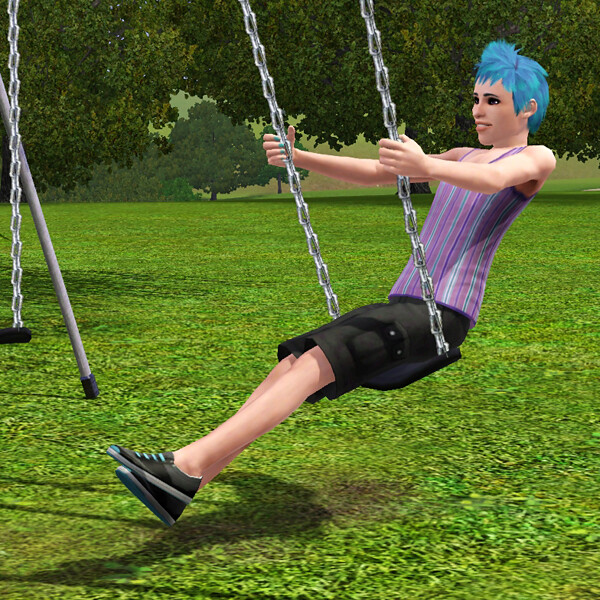The image is a hyper-realistic animation resembling a screenshot from a video game, likely The Sims, showcasing an avatar swinging on a swing set in a park. The central figure has a spiky blue pixie haircut, matching their bluish fingernails, and blue shoelaces on black shoes. They are smiling while swinging, wearing black shorts and a tank top with light blue, purple, and light purple stripes. The background features a manicured lawn with trees that appear to be a blend of painted and photographic elements, giving the scene an almost photographic realism. The avatar's proportions and features are noticeably animated despite the overall realistic appearance.